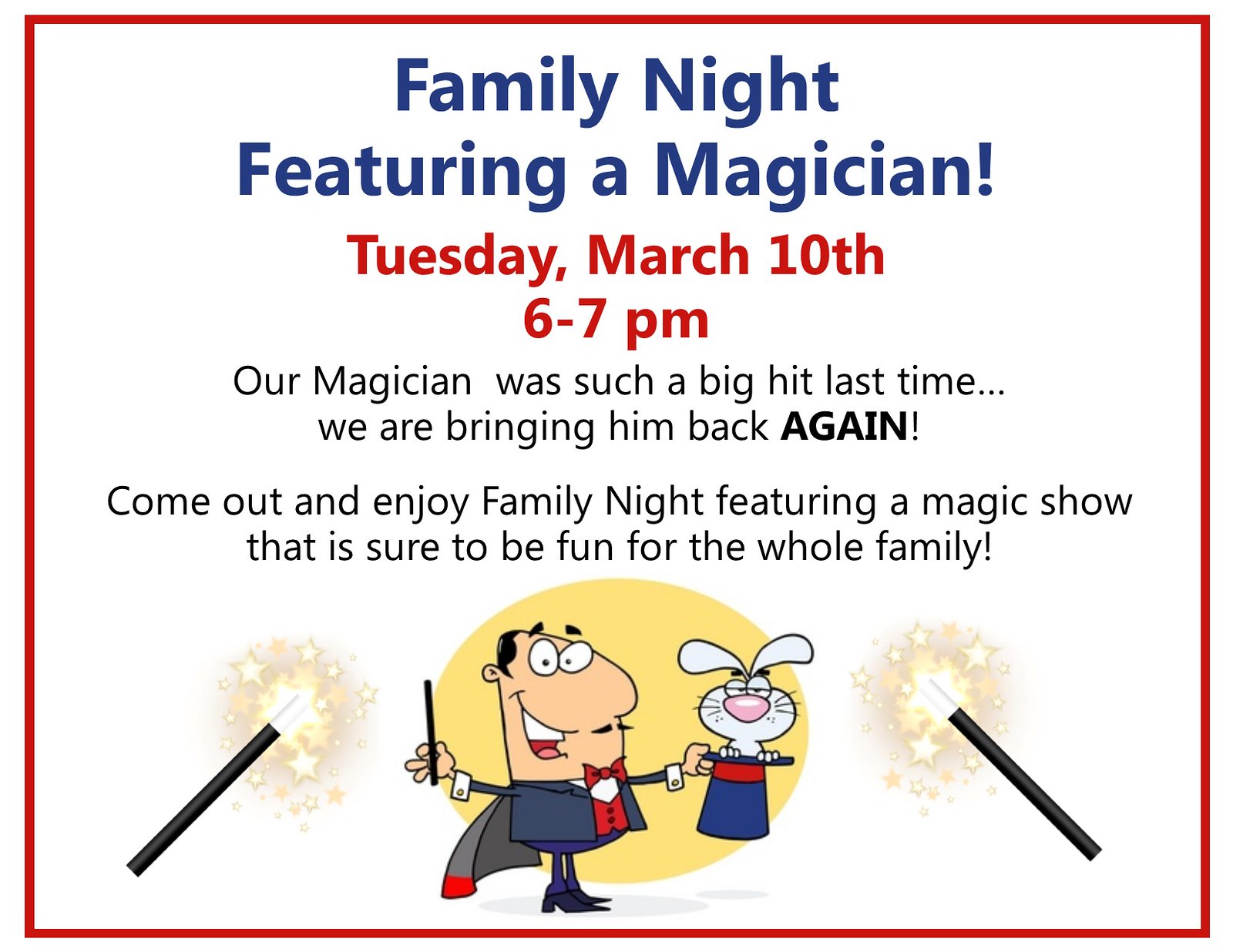The advertisement features a vibrant design with a solid red border surrounding a white background. At the top, bold, centered text announces "Family Night featuring a Magician!" scheduled for Tuesday, March 10th from 6 to 7 p.m. The text goes on to highlight that due to the magician's previous success, he is being brought back for another exciting evening. The poster invites families to enjoy a fun-filled magic show.

The lower part of the flyer showcases a colorful caricature of a smiling magician with dark hair, donning a cape, and performing classic tricks. In his right hand, he holds a magic wand, while his left hand presents a rabbit emerging from a blue top hat. The magician's image is set against a yellow oval backdrop, adding a touch of whimsical charm.

Enhancing the magical theme, the bottom left and right corners of the flyer depict animated black magic wands with white and golden starry tips. The overall color scheme includes red, white, blue, yellow, orange, gray, tan, and pink, making the advertisement visually engaging and appealing for family audiences.